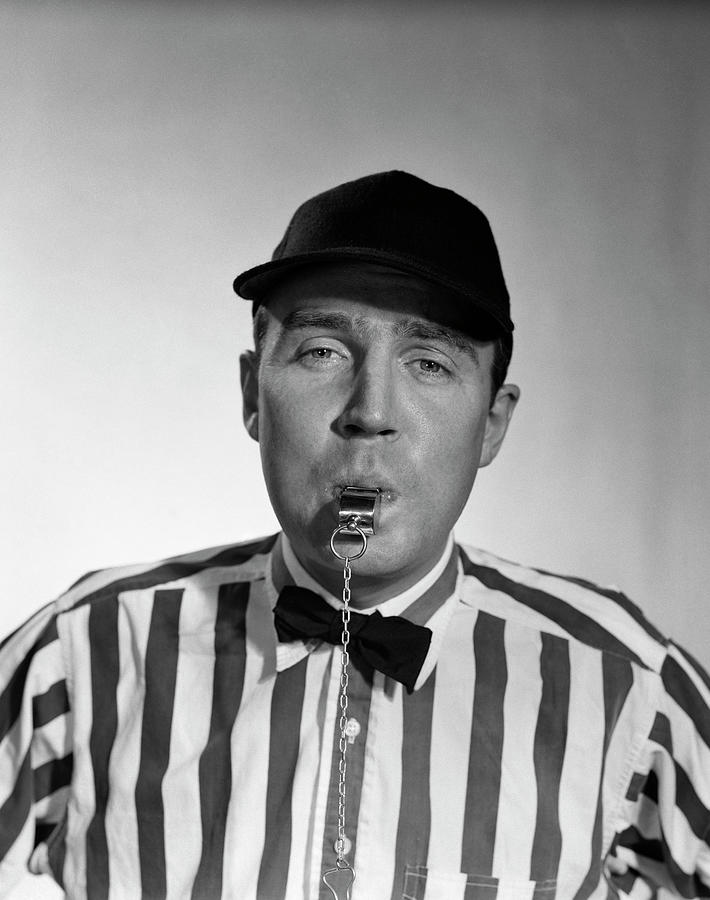This black-and-white photographic portrait features a serious-looking man dressed as a referee. He stands before a grayish background that transitions from lighter shades at the bottom to darker tones at the top right corner. He wears a black cap and a vertically striped button-up shirt with white and black stripes, which includes a front pocket and white buttons. At his neck is a black bow tie, and emerging from his mouth is a silver metal whistle attached to a chain loop. The man, who has thick eyebrows and partially closed eyes, appears poised to blow the whistle. The overall lighting suggests a professional, likely studio, setting, with some overexposure in the lower half of the image highlighting its artistic depth.